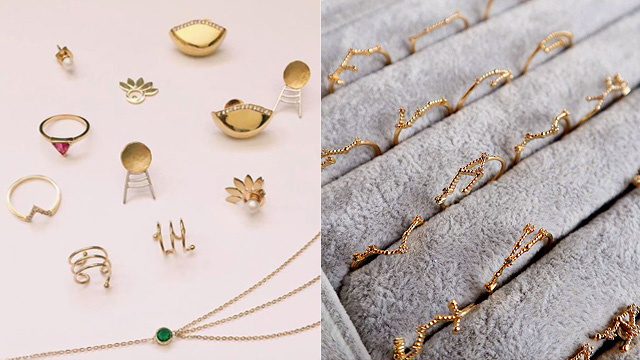This image comprises two distinct panels showcasing a diverse array of exquisite jewelry. On the right side, a soft gray, velvety display cushion features neatly aligned jewelry pieces. Here, gold bracelets, pendants, and necklaces adorned with shimmering diamonds are organized within the cushion's grooves, creating a refined presentation. There are no rings on this side, just an assortment of gold items with intricate diamond inlays, set against the plush gray backdrop.

On the left side, a lighter, almost pinkish surface serves as the backdrop for an assortment of more loosely arranged jewelry. This half includes a variety of gold items such as rings, a necklace with a central emerald, gold pins, bracelets, and brooches. A standout piece is a ruby ring with a large central gemstone surrounded by smaller diamonds. Additionally, a single pearl pin occupies the upper left corner of this panel, enhancing the overall elegance. There's also mention of small gold cups, likely intended for makeup, adding a unique element to the display. The jewelry here includes pieces with distinct features, such as a gold ring with diamonds inset around it, and a gold chain adorned with a green stone, possibly an emerald.

Overall, the image is a sophisticated exhibit of gold and gemstone jewelry, meticulously arranged for an eye-catching and detailed presentation.